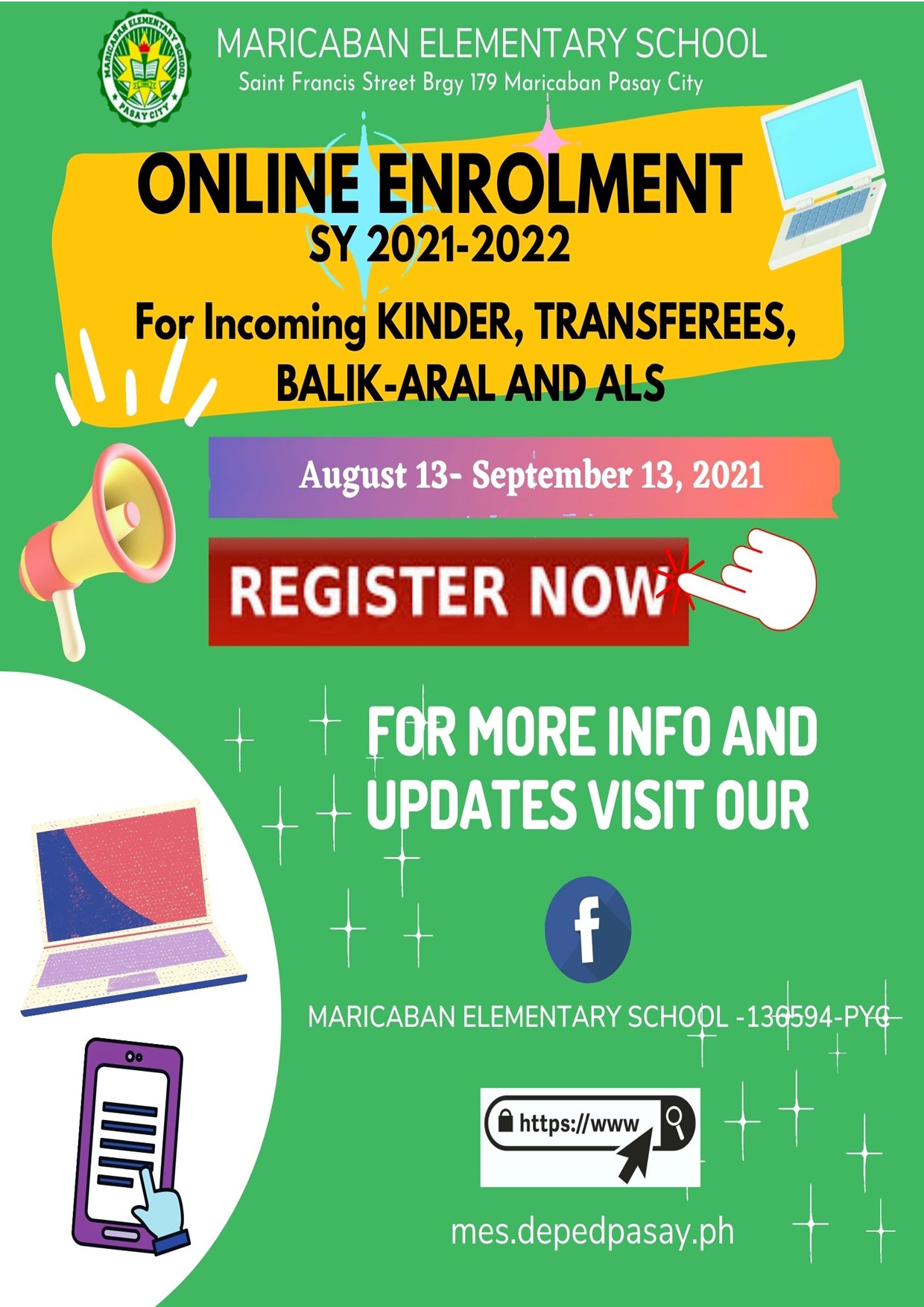**Detailed Caption:**

The image is a graphic poster promoting online enrollment for Maricaban Elementary School, located on St. Francis Street in Pasay City, Philippines. The poster is designed with an emphasis on engaging visuals and easy-to-read information. It announces the enrollment period for the academic year 2021-2022, specifically targeting incoming kindergarten students and transfer students. 

The enrollment period runs from August 13 to September 13, 2021, and potential enrollees are encouraged to register promptly. A call to action encourages people to visit the school's Facebook page for more information and updates, indicated by the Facebook logo and a link at the bottom of the poster.

The layout includes a variety of clip art images, such as laptops, a cell phone, and a loudspeaker, adding a modern and tech-friendly appeal to the design. The overall aesthetic of the poster is vibrant and appealing, aiming to capture the attention of parents and guardians looking to enroll their children.

The text is partly in Filipino, catering to the local audience, and the poster's domain ends in ".ph," confirming its Philippine origin.